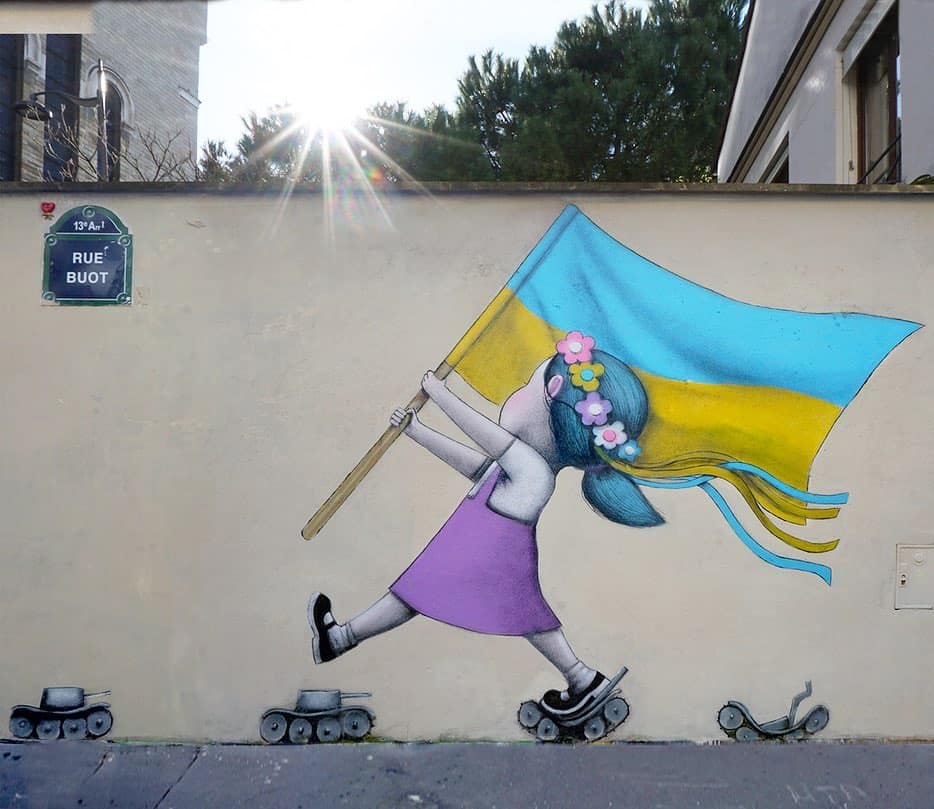The image is a photograph of a recent graffiti artwork on a beige wall in France, indicated by a black-on-white street placard at the top left that reads "Rue Buot." The mural vividly captures a small girl, her dark hair adorned with a vibrant garland of pink, yellow, purple, white, and blue flowers. Dressed in a purple dress over a white t-shirt, white socks, and black shoes, she marches defiantly while clutching a Ukrainian flag with its distinctive blue and yellow stripes. Her face is turned slightly away, revealing just her cheek. Below her feet, four Russian tanks line the street scene; the one farthest left is completely smashed, another is being crushed under her back foot, while her front foot hovers menacingly above the next. The scene exudes a sense of resilience and protest against the Russian government. Above the mural, sunbeams filter through trees, flanked by buildings and a visible light post, enhancing the artwork's dramatic effect.